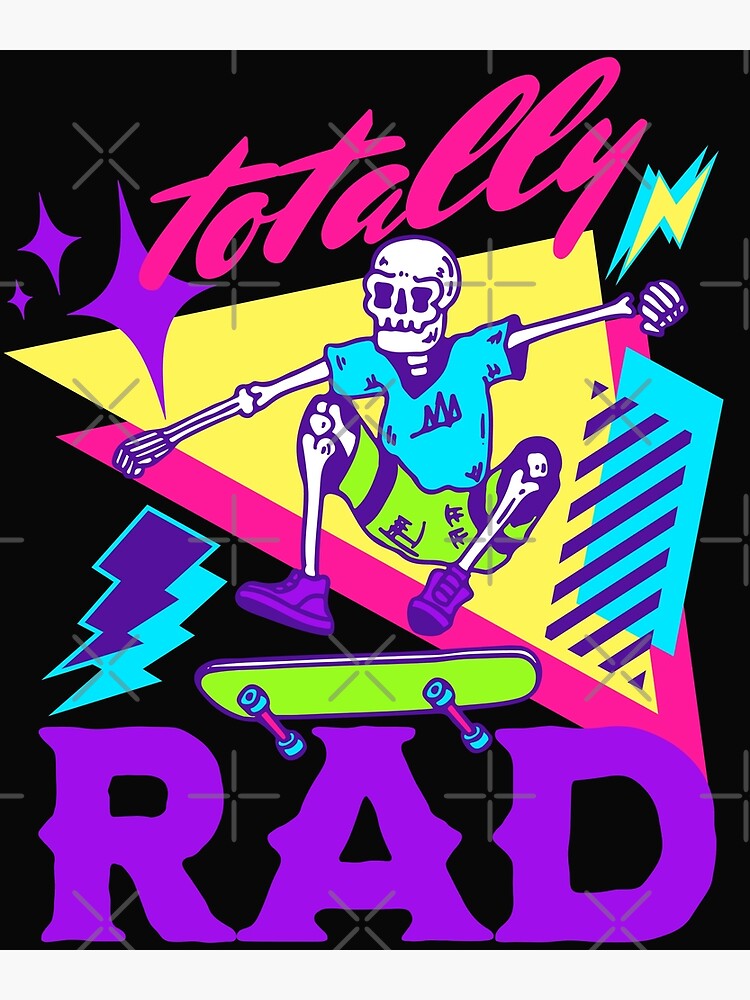The image is a vibrant, cartoon-style poster with a strong 80s and 90s nostalgia. At the center, a white skeleton outlined in blue is mid-jump above an electric green skateboard with blue wheels, evoking a sense of dynamic movement and action. The skeleton is stylishly dressed in a neon blue shirt, decorated with mountains, light green torn shorts, and purple tennis shoes. His arms are outstretched, and his legs are bent up as if performing a trick.

The background is a bold black, adorned with iconic 80s and 90s elements including neon and geometric shapes. Behind the skeleton, there's a layered yellow triangle over a pink triangle. Surrounding him are several neon symbols: three four-cornered purple stars, yellow lightning bolts, and a purple lightning bolt near his right shoe, with a dark blue striped box near his left shoe. 

The poster features the phrase "Totally Rad," with "Totally" in bright neon pink letters above the skeleton, and "Rad" in large neon purple letters under the skateboard. The overall effect is an explosion of electric colors and energetic shapes, encapsulating the skateboarding and stylistic vibes of the late 20th century.